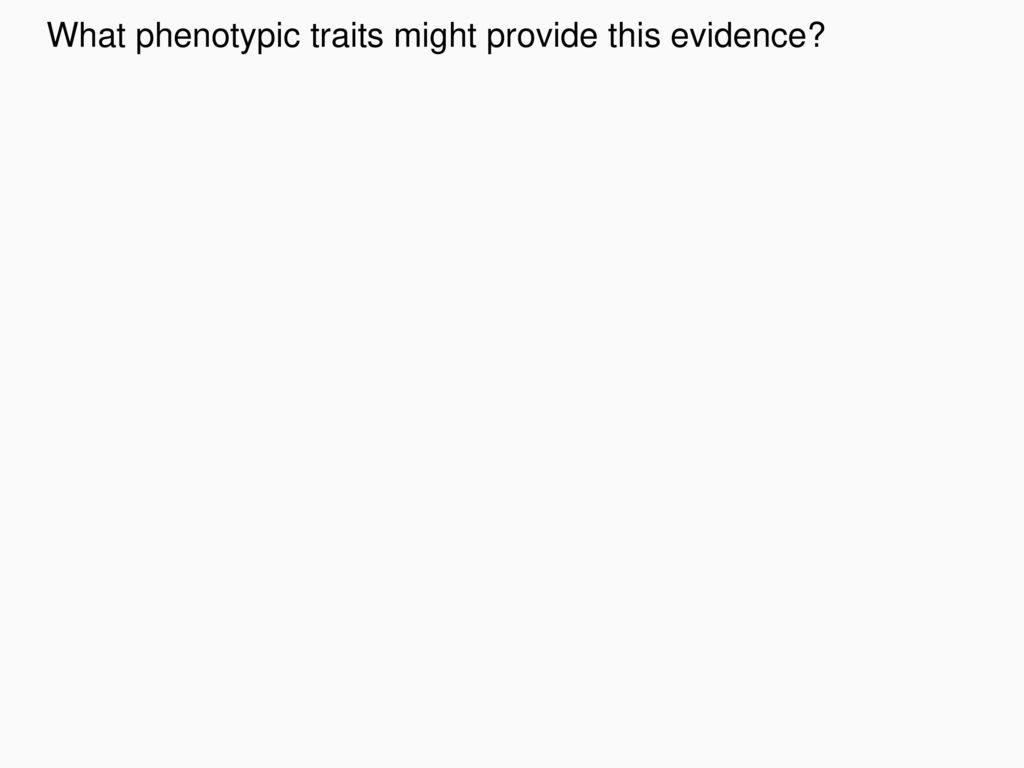A screenshot capturing a partial view of a webpage. The background is a very light gray, providing a neutral canvas. Dominating the top portion of the image, a single line of text in slightly larger, bold black font poses the question: "What phototopic traits might provide this evidence?" Below this query, the page is devoid of any additional text or imagery, featuring only the continuous light gray background, suggesting either an incomplete webpage or a section designed with minimal content. The absence of further elements lends a sparse and simplistic appearance to the screenshot.